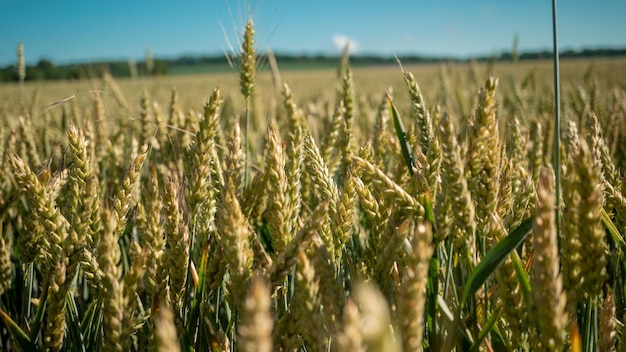This photograph captures an expansive field of yellow-colored wheat, likely on an American farm, such as one in Kansas. The wheat field stretches uninterrupted to the horizon under a bright blue sky, which has a few clouds dispersed. The image features a sharp focus on the individual stalks of wheat in the foreground, which appear to be mature and ready for harvest. Some green stems and leaves are also visible among the wheat heads, which have a long, silky appearance, almost resembling a woven pattern. As the field extends into the distance, the depth of field creates a soft blur toward the horizon, emphasizing the vastness of the landscape. There are no people, animals, or text in the scene, and a distant tree line subtly frames the background. Overall, the photograph conveys the serene and expansive atmosphere of a sunny, rural countryside.